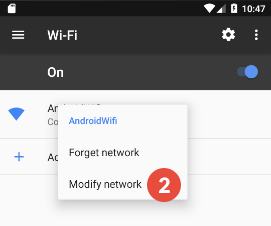The image depicts a smartphone screen showing the Wi-Fi settings interface. At the very top, various indicators such as the Wi-Fi signal strength, time, and battery status are displayed. Directly below these indicators, there are several icons and settings: a Wi-Fi label in white text, a circular gear icon for settings, and a three-dot menu button for additional options. A prominent "ON" button with a blue indicator is also visible, all set against a gray background with white text.

Further down, a section dedicated to Wi-Fi shows a blue indicator, signaling that Wi-Fi is active. An overlay pop-up window presents three options: “Android Wi-Fi” highlighted in blue, a "Forget Network" button, and a "Modify Network" option. Accompanying the "Modify Network" option is a red circular badge with the number 2, indicating notifications or additional settings.

In the background, there is a blue plus sign icon, suggesting the option to add another network. The top half of the image's background is black, transitioning to a white background on the bottom half, which displays various indicators and the pop-up for customizing wireless settings.